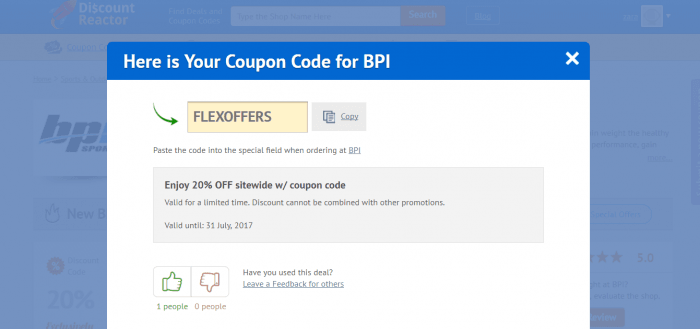Here's a cleaned-up and detailed caption for the image:

---

The image displays a coupon code for the online store BPI. The code provided is "FLEXOFFERS" in all capital letters. To use the code, copy it and paste it into the designated field during checkout on the BPI website to receive a 20% discount on all site-wide orders. This offer is valid until July 31st, 2017, and cannot be combined with other promotions.

The image also features green thumbs up and red thumbs down icons, asking users to provide feedback on their experience with the deal. Whether you liked it or not, you’re encouraged to leave a review for the benefit of other shoppers. Additionally, there is a convenient button that, when clicked, automatically copies the coupon code to your clipboard to ensure accuracy and ease of use.